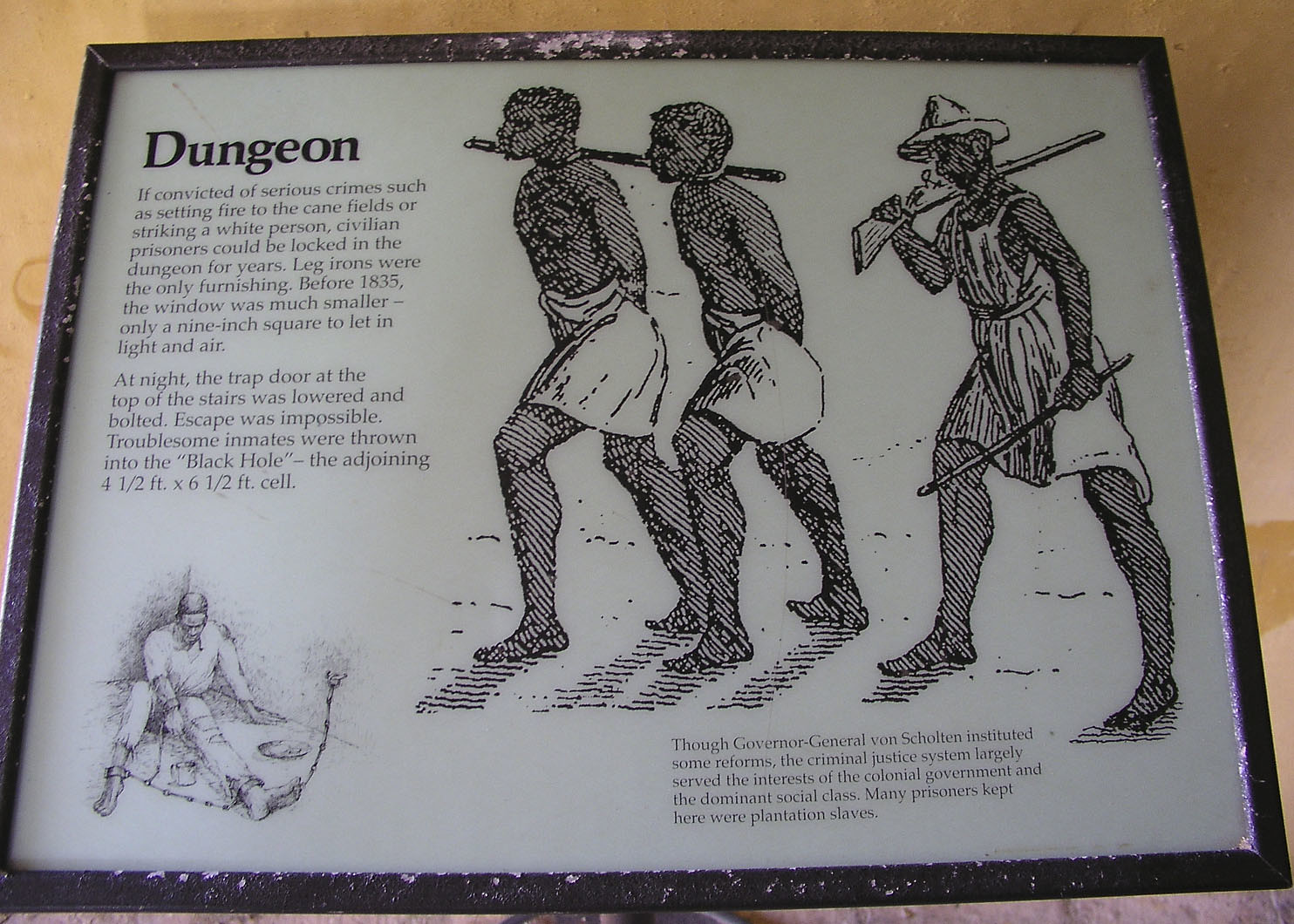This educational sign, framed in black and placed on a wall, features bold black letters on a white background. In the top left corner, it prominently displays the word "Dungeon". Below, dark text describes harsh punishments in the dungeon: "If convicted of serious crimes such as setting fire to the cane fields or striking a white person, civilian prisoners could be locked in the dungeon for years. Leg irons were the only furnishing. Before 1835, the window was much smaller, only a nine-inch square to let in light and air. At night, the trapdoor at the top of the stairs was lowered and bolted. Escape was impossible. Troublesome inmates were thrown into the black hole, the adjoining four and a half foot by six and a half foot cell."

The right two-thirds of the sign feature a detailed drawing. In the foreground, a man in a robe and hat is depicted with a rifle on his shoulder and a stick in his hand. He walks behind two topless, black men, whose hands are tied and who wear white skirts and are barefoot. The men are shackled by the neck to a rod held by the man with the rifle. In the lower left corner of the sign, a separate illustration depicts a black man in chains, wearing clothing and sitting with his head down. The chains bind his wrists and legs and are attached to the wall.

A caption complements the image: "Though Governor General Von Scholten instituted some reforms, the criminal justice system largely served the interests of the colonial government and the dominant social class. Many prisoners kept here were plantation slaves."